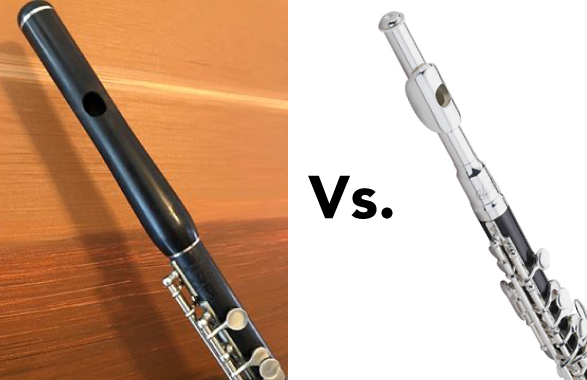The image features a detailed comparison of two flutes placed side by side against contrasting backgrounds. On the left, a sleek black flute with silver buttons is set against a light brown wooden backdrop, casting a noticeable shadow. This flute lacks the usual mouthpiece where air is blown. On the right, a shiny steel silver flute with black trimmings is displayed against a white background, highlighting the finger key areas more clearly. Between the two flutes, the word "VS." in black font emphasizes the comparison, possibly asking viewers to decide which flute is better or preferred. The photograph brings out the unique styling and intricate details of both the black and silver flutes, showcasing their similar slender designs and numerous metal buttons.